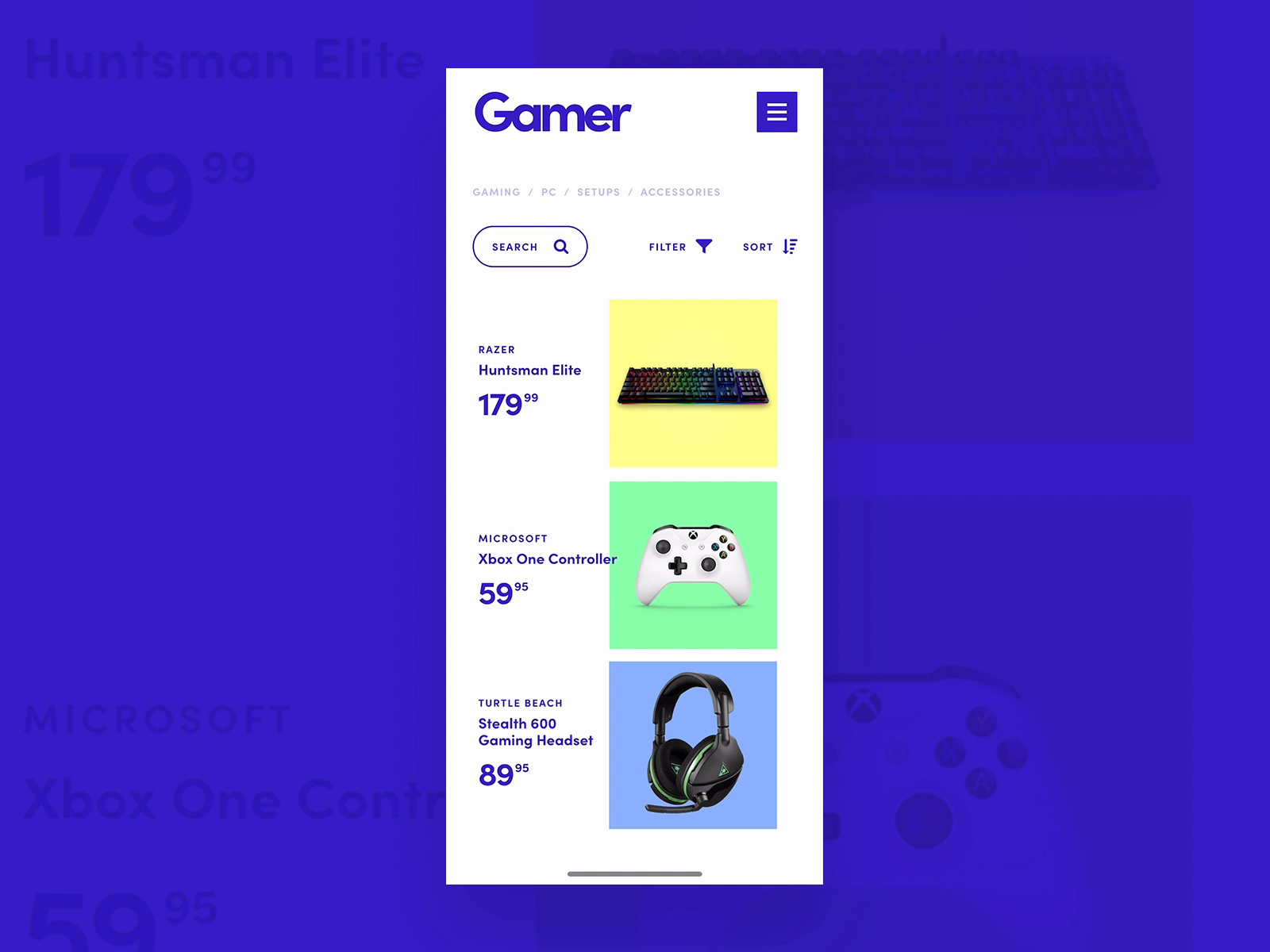The image displays a web page with a semi-transparent medium blue background. In the upper left corner, black text reads "Huntsman Elite" with a price tag of $179.99 below it. Adjacent to this text on the right is a picture of a keyboard. In the lower left, "Microsoft Xbox One controller" is listed with a price of $59.95, and to its right is an image of a white Xbox controller.

Overlaying the background is a prominent white box, approximately three times taller than it is wide. In the top left of this box, the word "Gamer" is written in blue text. In the upper right corner, there is a blue box containing three horizontal lines representing a menu icon.

Beneath the menu icon are three horizontally aligned menu options in smaller gray font: "Gaming," "PC," and "Setups and Accessories." Directly below, on the left, is a search bubble shaped in a horizontal oval containing the word "Search" and an accompanying magnifying glass icon. To the right are buttons labeled "Filter" and "Sort."

In the lower section of the white box are three images: a keyboard, an Xbox controller, and headphones. Each item is labeled on the left with its corresponding price.